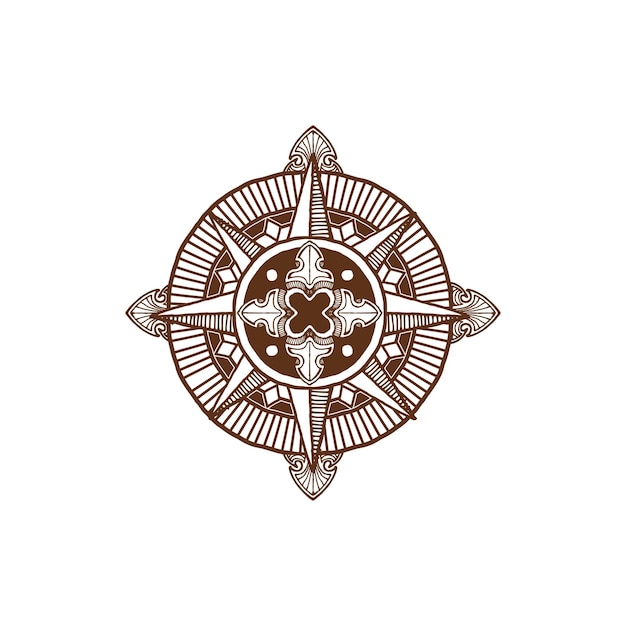This image features a detailed mandala-like design resembling a compass rose against a white background. At the center is a brown X with a white border, surrounded by four intricate arrow shapes that are reminiscent of inverted fleur-de-lis, all enclosed within a brown circle adorned with white dots. This central motif is bordered by a thin white line and an even thinner brown circle. Extending from this circle are eight triangles, each divided into a white left side and a right side with brown horizontal stripes. Encircling these triangles is another border decorated with small, pointed arrows in white and brown. Following this is a wider white border with brown lines, rounded off by an additional thin brown border. The outermost edge of the design features ornate, rounded arrow shapes. The overall palette is predominantly brown and white, evoking a sense of intricacy and traditional compass imagery, though the dominant brown may not appeal to everyone.